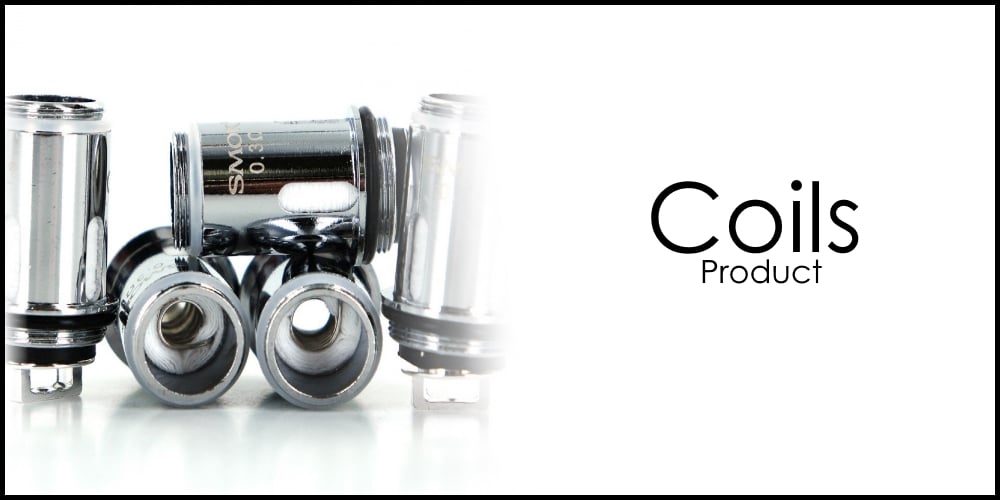The image appears to be a product advertisement featuring a central concept of "coils." The rectangular ad is framed by a thin black border and set against a white background. On the right side of the ad, bold black text reads "COILS," with smaller subtext below stating "PRODUCT." 

The left side showcases a detailed photograph of five cylindrical, shiny metallic coils, which appear to have a plastic and metal base. The coils are potentially mechanical or electronic devices, possibly components of larger systems like faucets or pipes, given their threaded ends. The arrangement is as follows: two coils are standing upright on the left and right ends of the image, while two others lie side-by-side horizontally in the middle. A fifth coil is positioned perpendicularly on top of the middle two. The coils' shiny, chrome-like surfaces reflect light, enhancing their metallic appearance. Some visible markings on the coils read "SMO 0.30," adding to the product details.